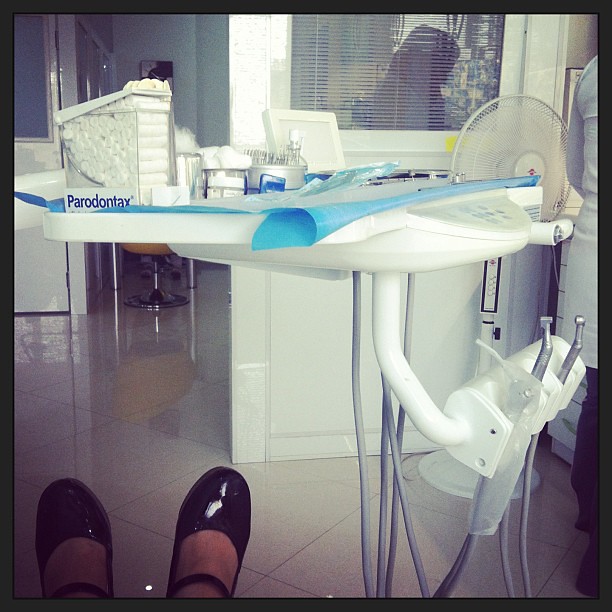This photo captures the perspective of a patient seated in a dentist's chair, with their legs extended and feet, clad in black patent leather shoes, visible at the bottom left of the frame. Dominating the foreground is a white tray table laden with dental instruments, gauze in a clear container, and possibly a blue bib. The tray also holds various dental tools and tubes, suggesting readiness for a dental procedure. The backdrop features an office space with off-white or light green walls, a fan, and vertical blinds. Behind the blinds, a shadowy silhouette of a woman, likely another patient or staff member, can be discerned. To the right edge of the frame, a hint of a doctor in a white coat can be seen, adding to the clinical atmosphere of the scene. The floor is a reflective grayish-white, contributing to the sterile environment typical of a dental office.